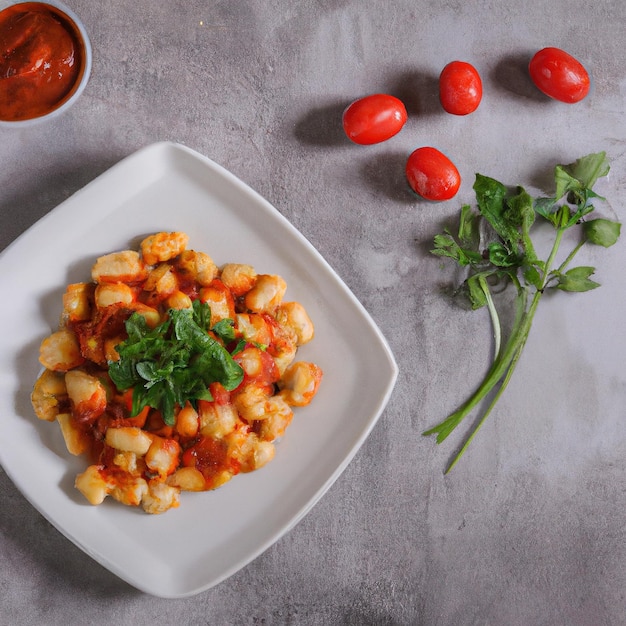The photograph features a carefully styled food presentation set against a pale gray, cement-like background, which could be either a countertop or table setting. In the upper left corner, a small round dish contains a thick, dark red sauce, possibly ketchup or chili sauce. The upper right corner showcases four bright cherry tomatoes alongside a sprig of fresh green garnish, likely basil or parsley. Dominating the center of the image, a white square plate with raised edges holds a neatly stacked dish that could be composed of either crab, meat, or potato tops, generously drizzled with the same red sauce and topped with finely chopped green herbs, adding a touch of elegance to the arrangement.